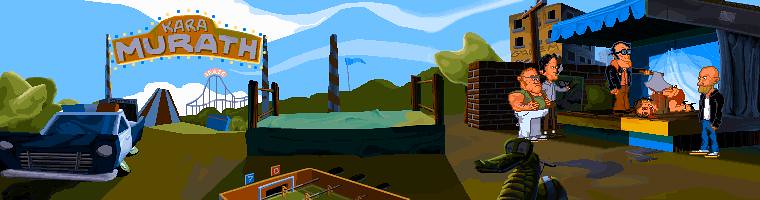The image appears to be a detailed, unsettling cartoon scene, possibly from a game. The setting includes a stage with a blue canopy, where a man in a black coat and glasses stands holding an axe embedded in the back of a person lying prone on the stage, bleeding profusely. Surrounding this stage are five other individuals. One, apparently very angry, stands beside the stage, while two others in front exhibit annoyance or indifference—one man is smoking. Another man in a black and white coat, who is bald, stands nearby, alongside a man in a green sleeveless shirt with glasses and another in a blue button-up shirt with brown pants.

The backdrop features a dilapidated, multi-story building with no glass in its windows and unreadable writing. A partly visible red brick wall with white mortar stands between this building and the stage. Further back, a sign reads "Kara Marath," and there is a flag, a roller coaster, and a red and white tent suggestive of carnival elements. A black and white police car with a crooked tire, a foosball table, and a toy-like alligator for rocking are scattered in the middle ground. The right side of the image shows a brown wrestling ring with a white mat missing some ropes, adding to the chaotic environment. The sky background is a baby blue with white waves mimicking clouds, completing the surreal and detailed setting.